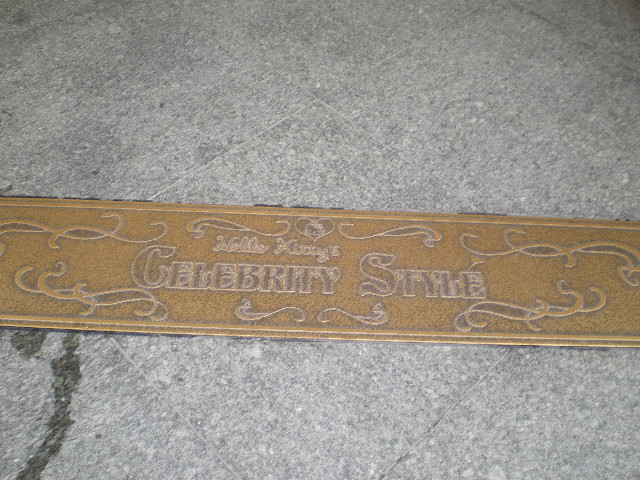This image captures a close-up view of a rectangular, bronze-colored plaque embedded in a large, stone tile walkway, likely at the entrance of a shop. The walkway is made up of somewhat empty, large gray and tan concrete tiles, each about three feet by three feet. The centerpiece of the photo, the plaque, runs horizontally across the middle of the image. The plaque itself features intricate designs and a heart logo above the prominently etched words "Hello Kitty's Celebrity Style," with each word capitalized. The lettering, lighter than the plaque's golden bronze hue, stands out against the detailed backdrop. This outdoor setting, bathed in natural light, makes for an elegant entrance marker.